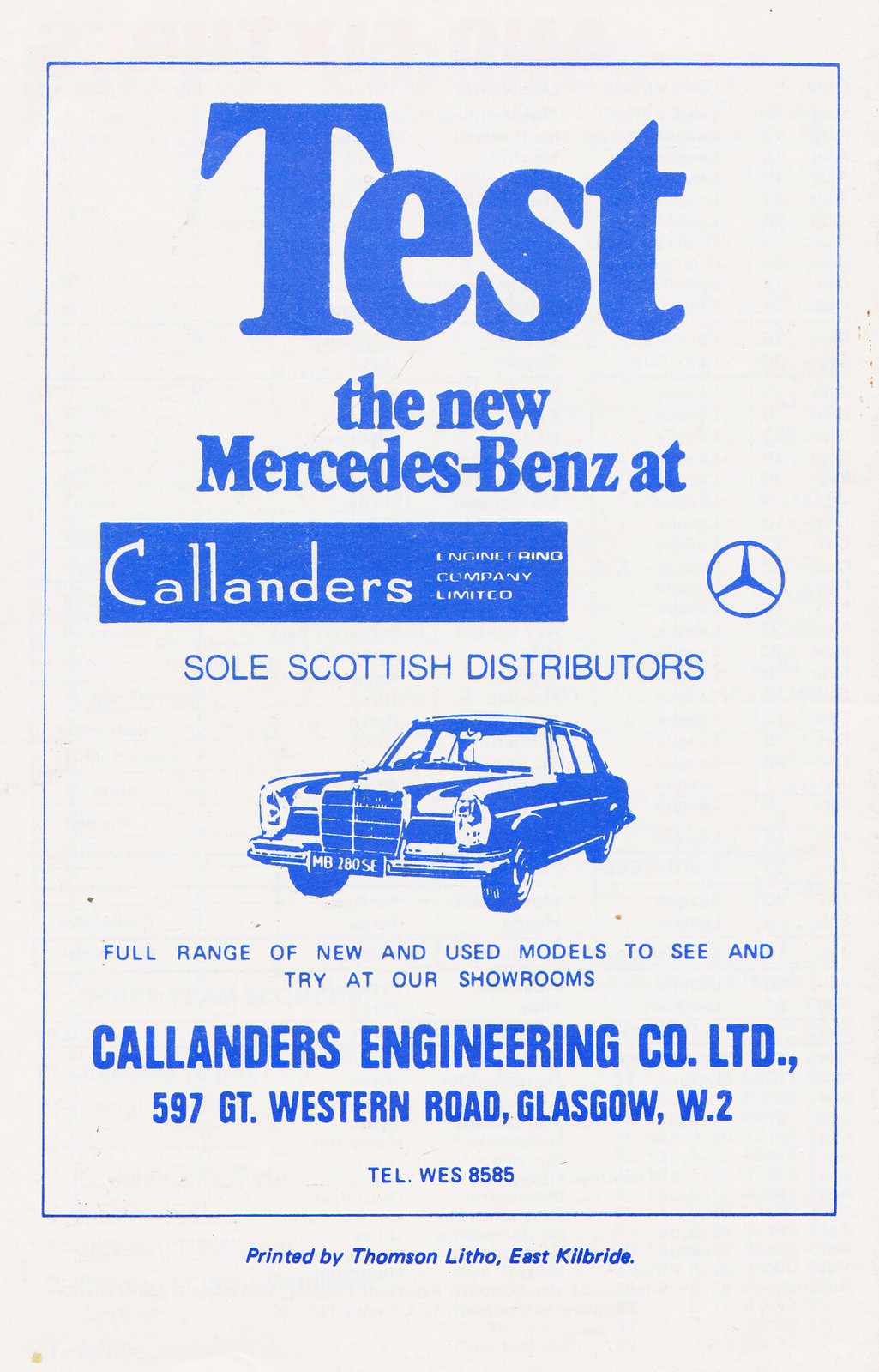This is a detailed advertisement flyer for Mercedes-Benz, printed on off-white paper with blue text. The highlight of the flyer is the large, bold word "Test" at the top, followed by the phrase "the new Mercedes-Benz at Calendars." It prominently features the Mercedes-Benz logo and declares "sole Scottish distributors." An intricate sketch of a vintage Mercedes-Benz vehicle is displayed underneath this text. The flyer advertises a "full range of new and used models to see and try at our showrooms," with the name "Calendars Engineering Co. Ltd" in a bold blue font. The address "597 GT Western Road, Glasgow W2" and telephone number "WES 8585" are clearly provided. A blue border frames the entire layout, and the flyer notes at the bottom, "Printed by Thompson Litho, East Kilbride."